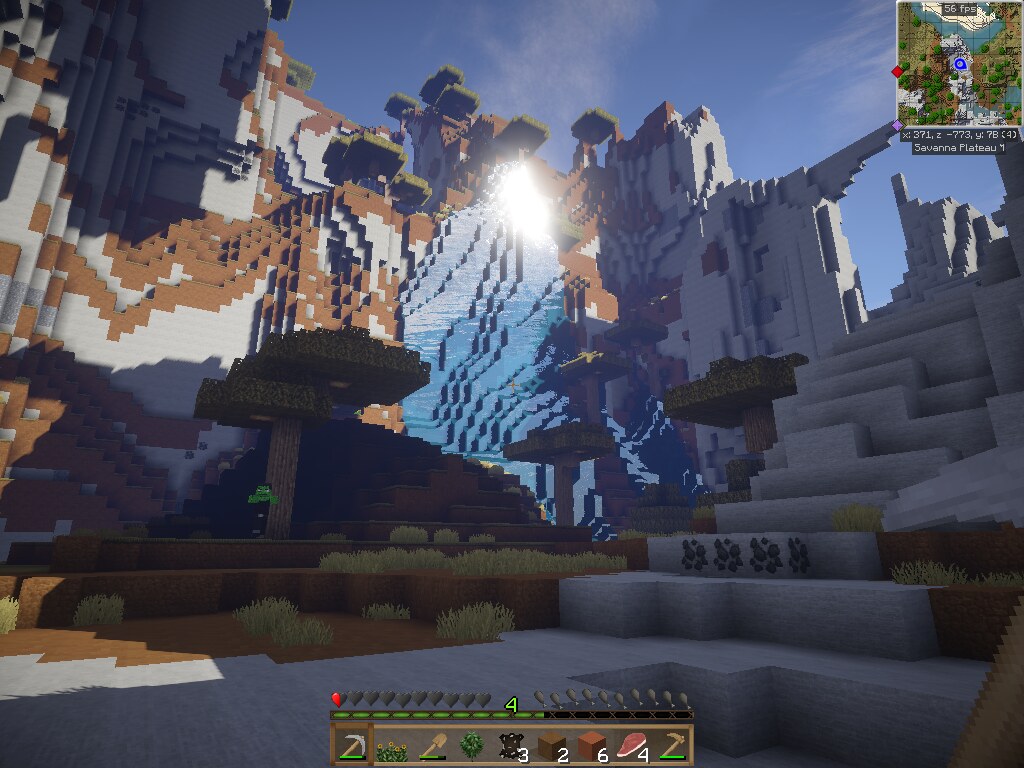This image depicts a meticulously designed Minecraft scene featuring a stone sculpture. On the right-hand side, white steps ascend in a straight path, leading to an elegant arch bridge that spans above them. The left-hand side is populated with a variety of blocky trees, each with vibrant green canopies. Amid the trees, reddish-brown steps, possibly made of mud or dirt blocks, create a rustic path that leads towards the central structure.

A striking blue waterfall cascades down, forming a river that flows through the scene, adding a dynamic element to the tranquil setting. The top portion of the image is radiant, reflecting sunlight from an unseen source, adding a gleaming brightness that enhances the overall visual appeal.

To the left, there appears to be a castle-like structure, predominantly white with brown accents. This castle, possibly part of a virtual tour, stands out distinctly within the natural and crafted elements of the scene. The combination of architectural and natural elements creates a harmonious and captivating Minecraft landscape.